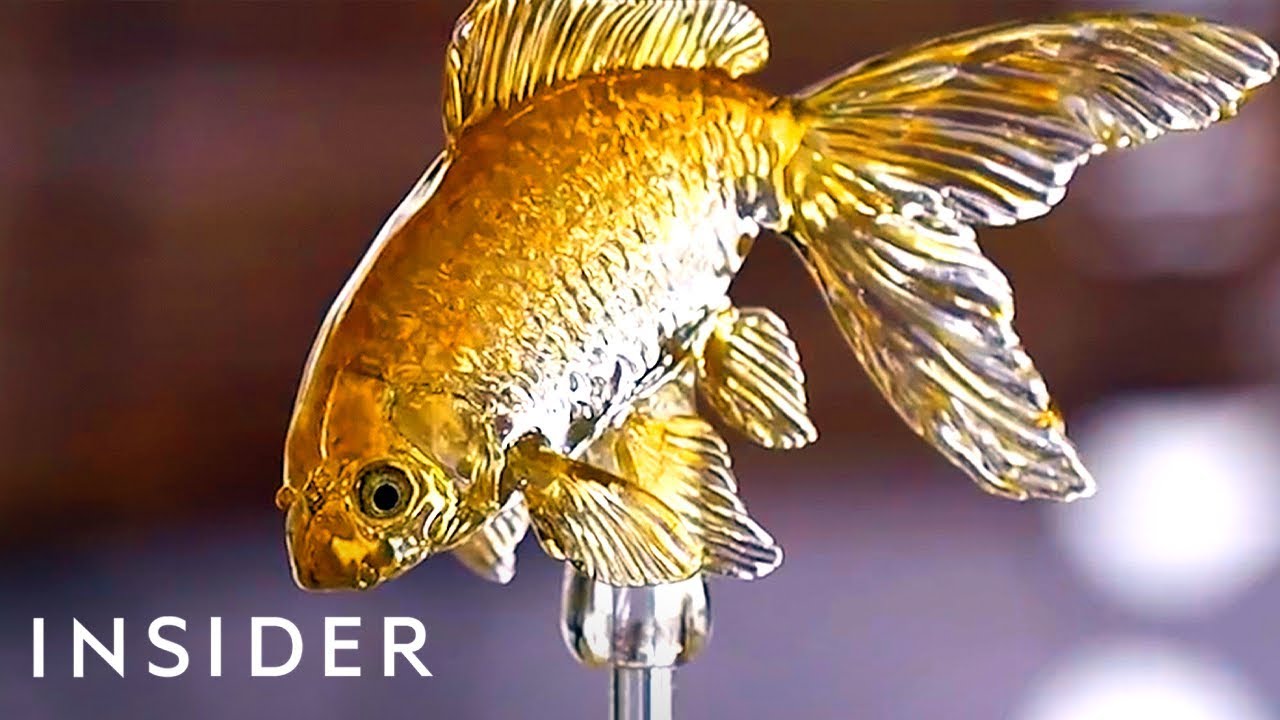The image features an intricately detailed glass or plastic sculpture of a goldfish perched atop a sleek, silver metallic pole. The fish exhibits pronounced features including a large tail fin, a prominent dorsal fin, pectoral fins, and a detailed texture showcasing its scales and black pupils. The transparent fins and overall shiny, orangish-golden hue add to its lifelike yet artistic appearance. In the blurred, dark grayish or purplish-brown background, white lights are faintly visible, adding a subtle contrast. Prominently displayed in the lower left corner is the word "INSIDER" in bold, white capital letters, suggesting the image may be part of a magazine or article.